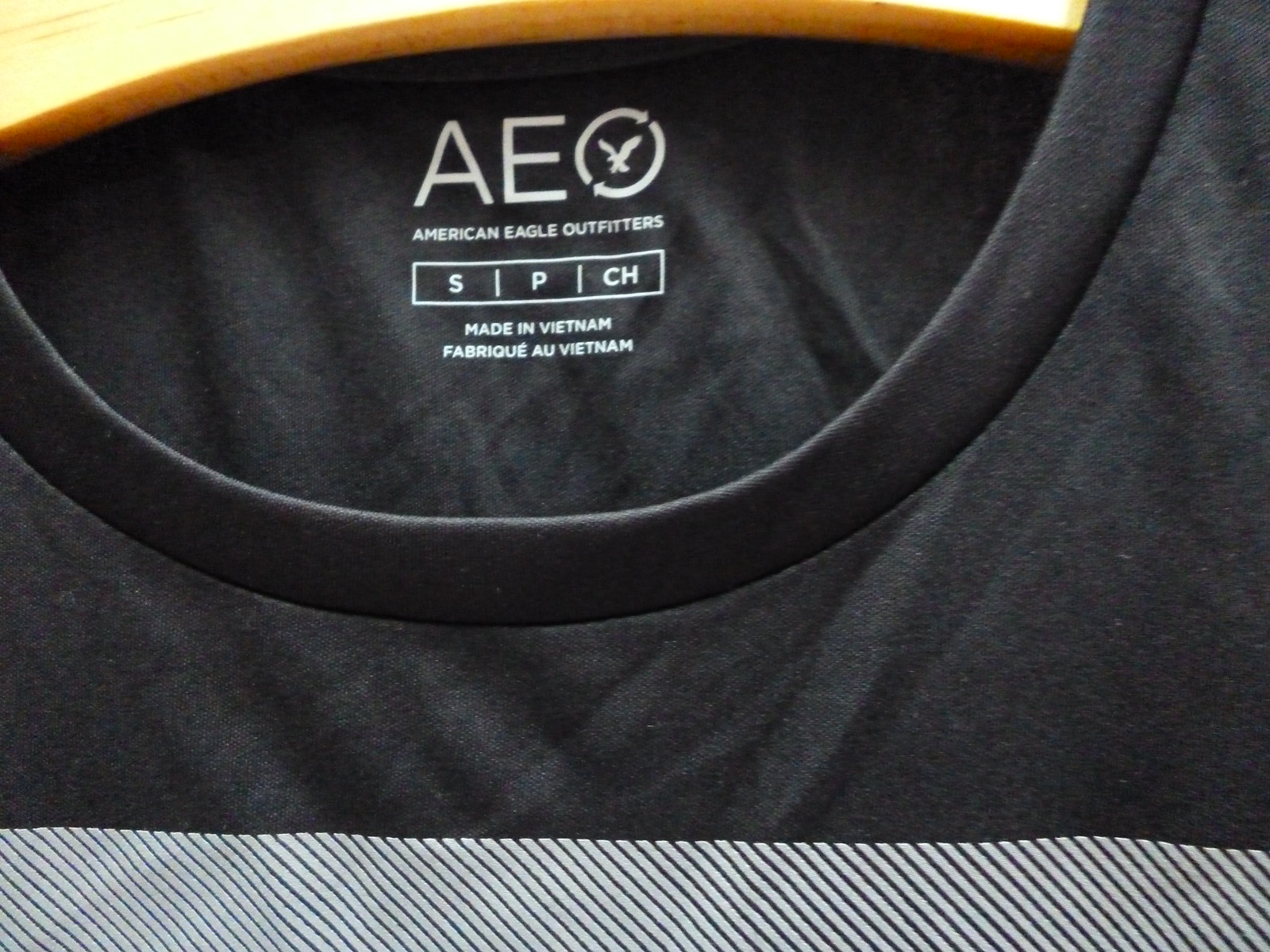This close-up photograph captures a dark gray, almost black t-shirt from American Eagle Outfitters, focusing on the printed label at the neckline. The shirt is displayed on a wooden hanger, visible at the top of the image. The label, printed in white font directly on the fabric, prominently features the brand's initials "AEO" with a silhouette of a flying eagle inside the "O." Below this, "American Eagle Outfitters" is clearly written. Further down, information about the shirt's size appears, marked as "S," "P," and "CH" within a segmented rectangle. The label also notes the shirt's origin with the text "Made in Vietnam" followed by its French equivalent, "Fabrique Vietnam." Just beneath the label area, the t-shirt transitions to a pattern with horizontal stripes in light gray or white, alternating with stripes in dark gray or possibly dark green.